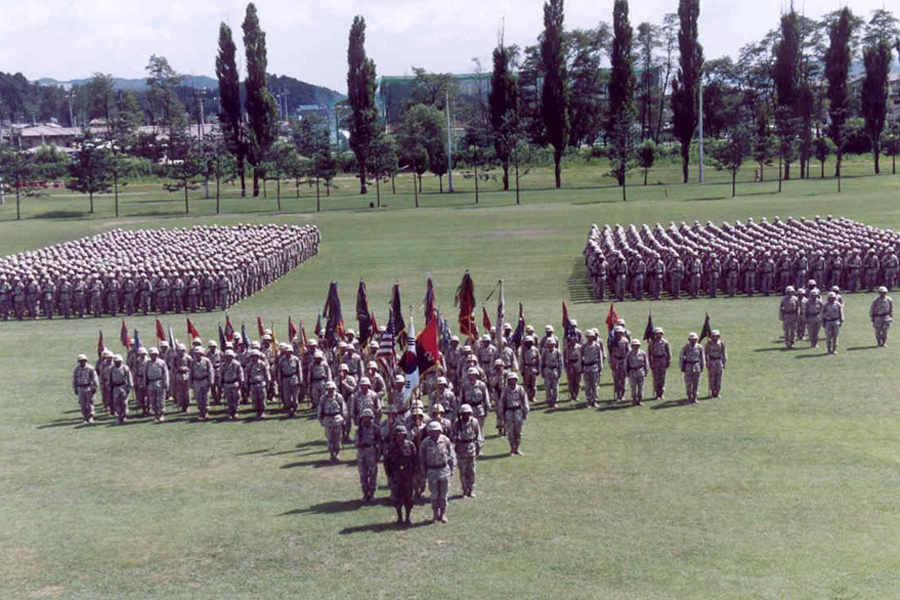In the image, we observe a large number of soldiers participating in a ceremonial event on a sprawling green field that occupies the majority of the lower portion of the picture. The soldiers are arranged in several distinct formations. To the left and right, there are solid squares of soldiers lined up in precise rows, extending into the distance. Near the center, a smaller group of soldiers is arranged in an arrow-shaped formation, with some elements resembling a star, marching forward. Leading this central group are soldiers bearing multiple flags. In the background, there are very tall trees with lush green leaves, creating a natural border. Further in the distance, the horizon is dotted with white shapes of houses and a notable tall building with a green color and flat rooftop, amidst white clouds. The scene captures the disciplined coordination of what seems to be an army or military group, possibly consisting of 200 to 300 individuals.